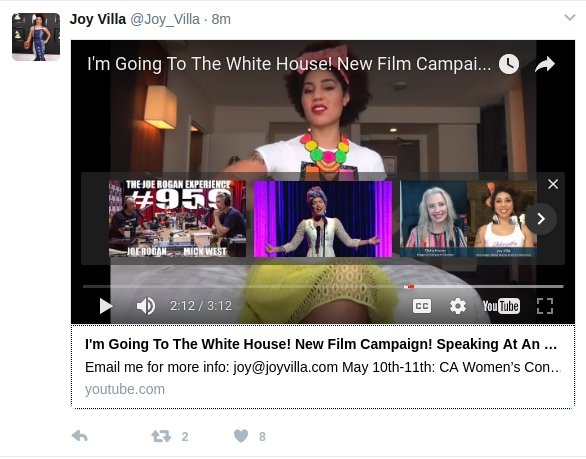This screenshot captures a recent social media post made by Joy Via, identified by her handle @joy_via, just eight minutes prior. Joy shares an announcement about her new YouTube video, enthusiastically titled "I'm going to the White House! New Film Campaign!" The video's timestamp reveals it to be 3 minutes and 12 seconds long, though the screenshot pauses at 2 minutes and 12 seconds, suggesting a specific segment of the video being highlighted.

In her post, Joy encourages viewers to email her at joy@joyvia.com for more information. Additionally, she mentions speaking at the CA Women's Conference, scheduled for May 10th or 11th, aligning with the video's apparent promotional content.

The standard YouTube interface is visible, including options like watch later, share, play/pause, volume control, closed captions, settings, a direct link to YouTube, and fullscreen mode, underscoring the platform’s interactivity features.